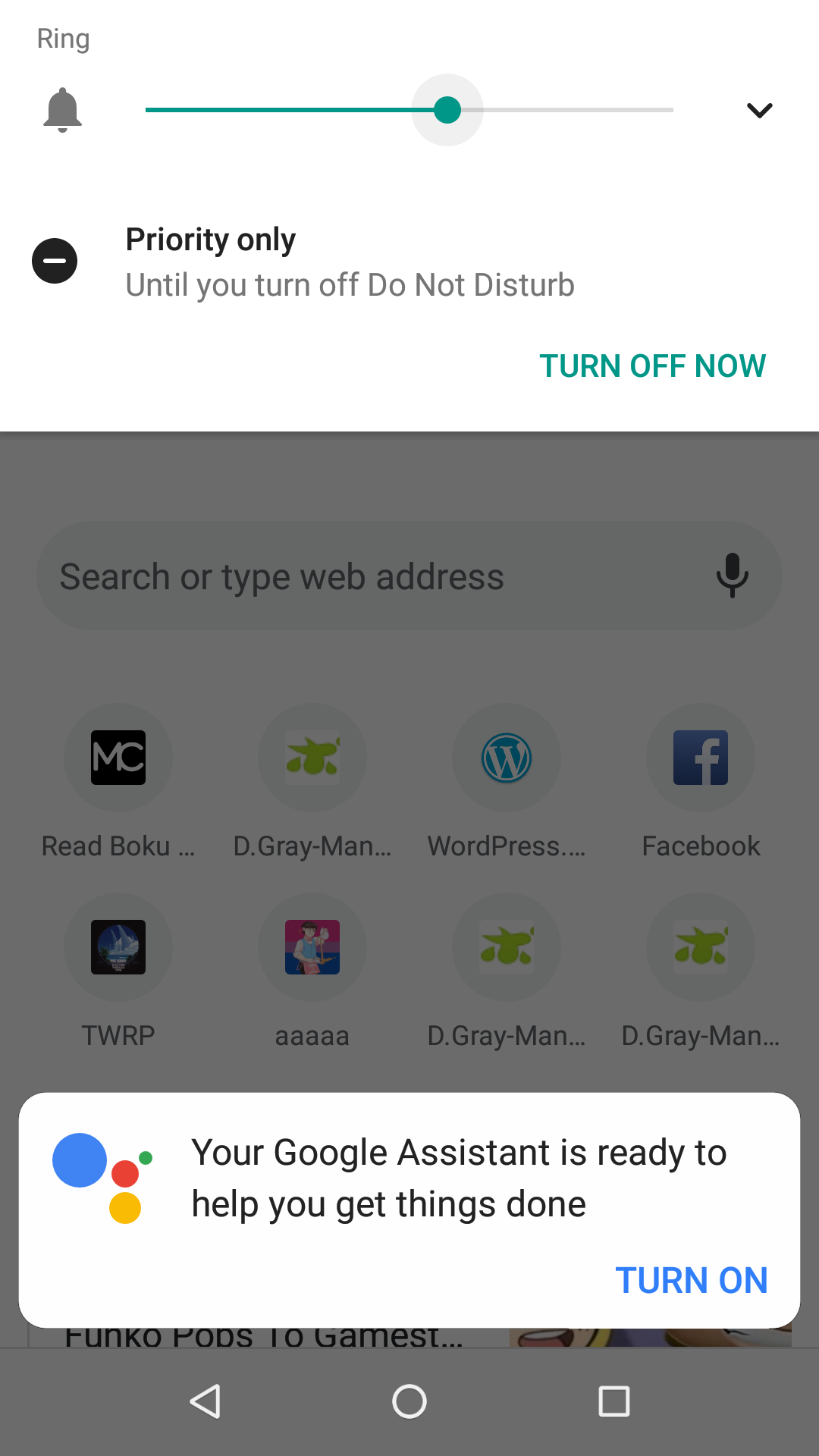The image features a detailed illustration with a white background at the top. On the left side, there is the word "Ring" accompanied by a small bell icon. A green line extends vertically from this section, leading to a green dot situated slightly over halfway down the line. Below the dot, a downward arrow is visible, followed by a black circle containing a white minus sign, and the text "Priority only until you turn off Do Not Disturb" is displayed next to it. Below this, in green text, it says, "Turn off now."

The lower half of the image transitions into a gray background with a white box at the top. Inside this box, there's a large blue circle accompanied by smaller circles in red, yellow, and green. The text within this section reads, "Your Google Assistant is ready to help you get things done." Below this text, there is a blue button labeled "Turn On."

At the very bottom of the image, the design returns to a gray background containing a bar with a triangle, circle, and square, which represent navigation buttons.

Overall, this illustration provides step-by-step instructions on how to disable the Do Not Disturb feature while highlighting the assistance offered by Google Assistant.